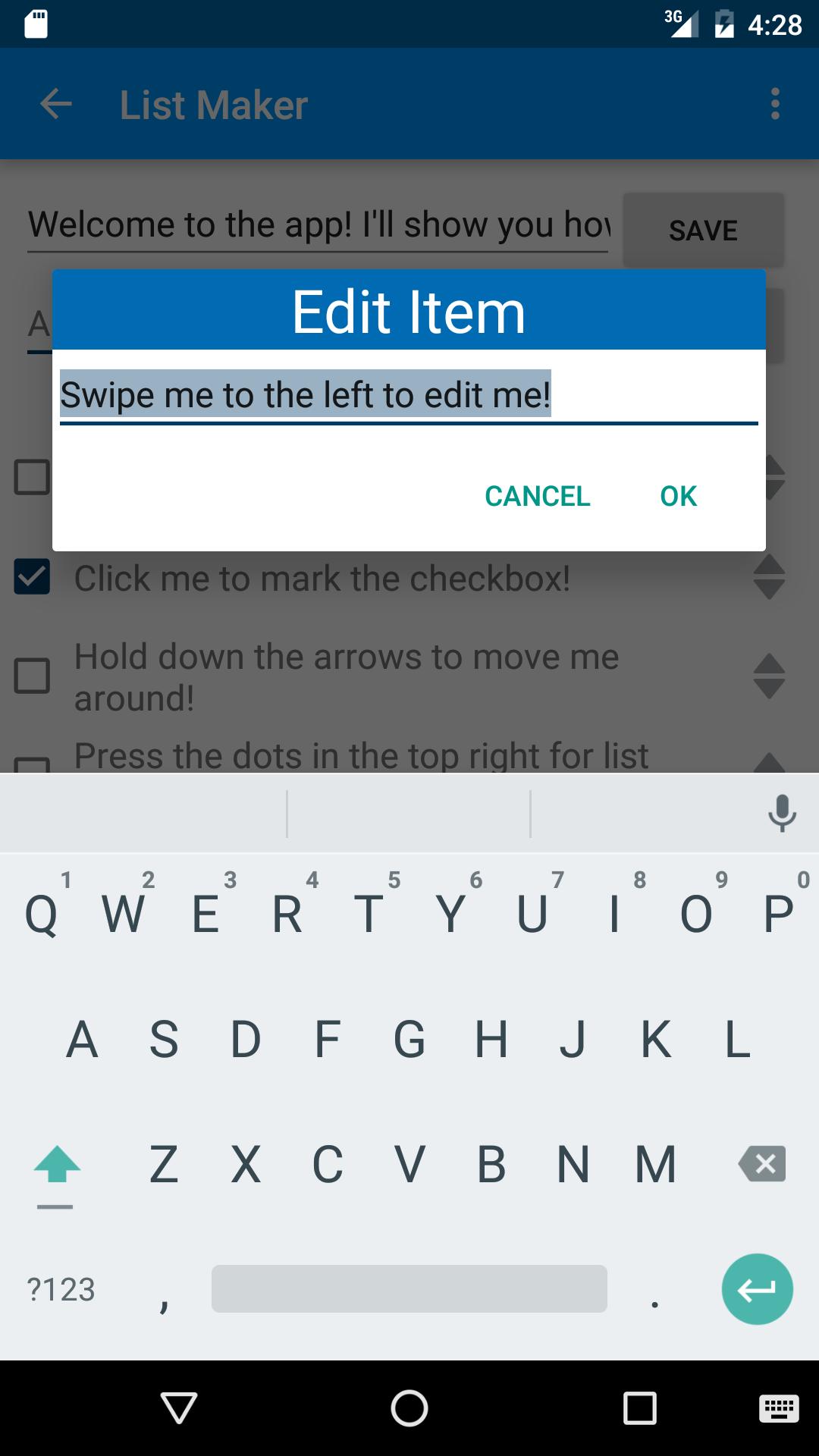The screenshot captures an editing interface of a mobile application called "List Maker." The top right corner of the screen shows device-related information: the battery icon (charging and halfway charged at 4:28), network signal (3G), and status bar elements on a light gray background. Below this, a blue header bar displays the title "List Maker."

Under the header, text welcomes the user to the app and provides instructions: "I'll show you how." A gray "Save" button is also visible. A rectangular prompt obscures part of this text, showcasing a user action guide that reads, "Click me to mark the checkbox," where the checkbox is currently marked. The instructions continue with tips saying, "Hold down the arrows to move me around, press the dots in the top right for the list."

A central dialog box titled "Edit Item" appears prominently, containing a text input field with the instruction "Swipe me to the left to edit me." This text is highlighted in gray, indicating it is selected. Below the input field are two actionable buttons: "Cancel" on the left and "OK" on the right, both in blue text.

The bottom portion of the screen displays the standard QWERTY keyboard layout. At the very bottom, a thin black bar features navigation icons: an upside-down triangle, a circle, a square, and a keyboard icon located in the bottom right corner.